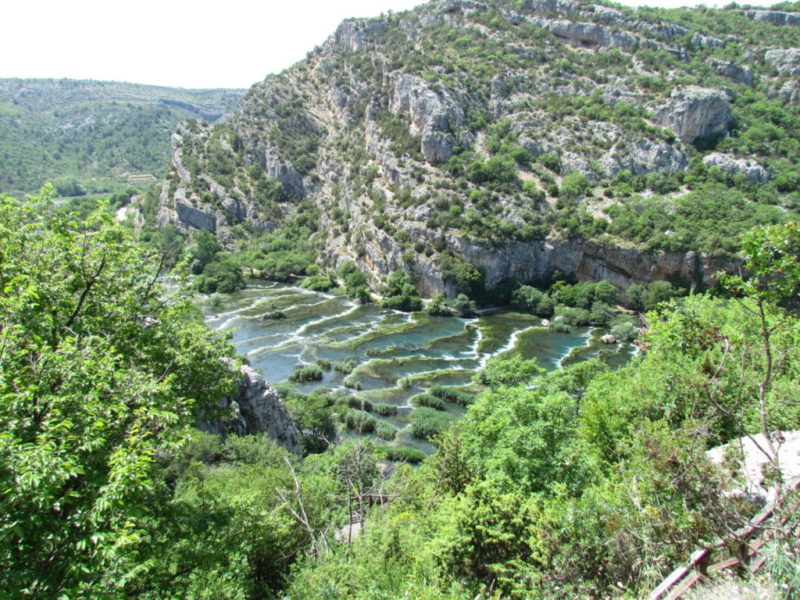The photograph, measuring approximately 9 inches by 9 inches, captures a vast, mountainous landscape, possibly located in South America, with an emphasis on a river and waterfall that cascade down through varying levels in the center of the image. Lush, green trees populate the mountains, stretching up the hillsides, and the lower areas feature scrubby vegetation and rocky outcrops. The scene appears to be taken from a vantage point atop another mountain, providing a view of the opposite hillside, which is also forested. The water body flows amid the greenery, possibly a flood plain, with tree tops emerging from the water. The bright daylight sky is prominently white, likely due to the photo's exposure or a hazy atmosphere. The bottom right corner of the photo includes additional scattered trees and rocky formations. Overall, the image intricately details a rich natural environment, filled with diverse plant life and dynamic water movement, set against a rugged mountainous backdrop.